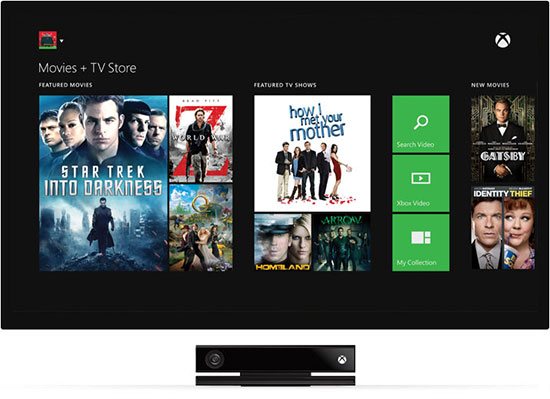This screen displays a digital movie and TV store interface, featuring a sleek black background. On the upper left corner, there is a square whose click reveals a pull-down menu. Adjacent to it, there's a circular icon with an X through it—likely indicating the Xbox platform. To the immediate right, in prominent white text, it states "Movies + TV Store."

Beneath this heading, a section titled "Featuring Movies" showcases titles including "Star Trek Into Darkness," along with a partially obscured title that appears to include "WR" and a Z, indicative of "World War Z." Another small, indistinct movie title appears nearby but its specifics are unreadable.

To the right, under the banner "Featured TV Shows," titles listed include "How I Met Your Mother," "Homeland," and "Arrow." Below these titles, there are three vertically stacked orange boxes labeled "Search Video," "Xbox Video," and "My Collection."

Further down on the right, under the heading "New Movies," notable titles include "The Great Gatsby" and "Identity Thief."

At the bottom center of the screen, there is a long black rectangular bar. On the right end of this bar is another icon featuring a circle with an X, reflective of the Xbox logo. To the left end, there appears to be a watermark resembling an eye.